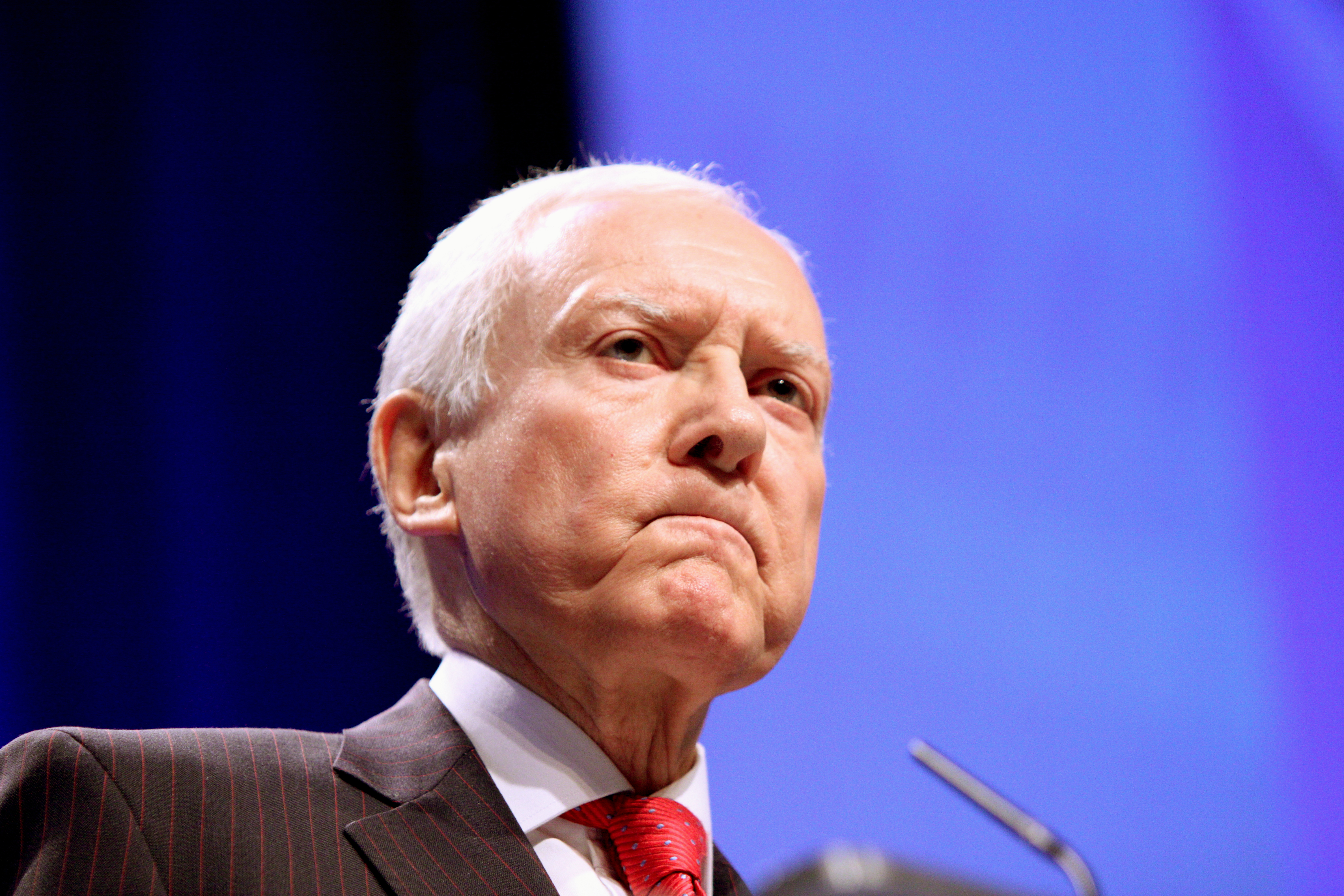This photographic image captures an older white man, likely in his 60s or 70s, distinguished by a receding hairline and gray hair. Dressed in a gray suit, white shirt, and red tie, he stands indoors, likely at a podium, and is partially obscured by a gray microphone. His expression is somber, with his mouth turned down in a frown as he gazes slightly away from the camera, toward the top right corner of the frame. The background features a split screen, one half black and the other half light blue with a purple streak, suggesting a projection or slide presentation. His demeanor and formal attire, along with the setting, suggest he might be an executive or a politician addressing an audience, and he appears displeased or concerned about the situation at hand.